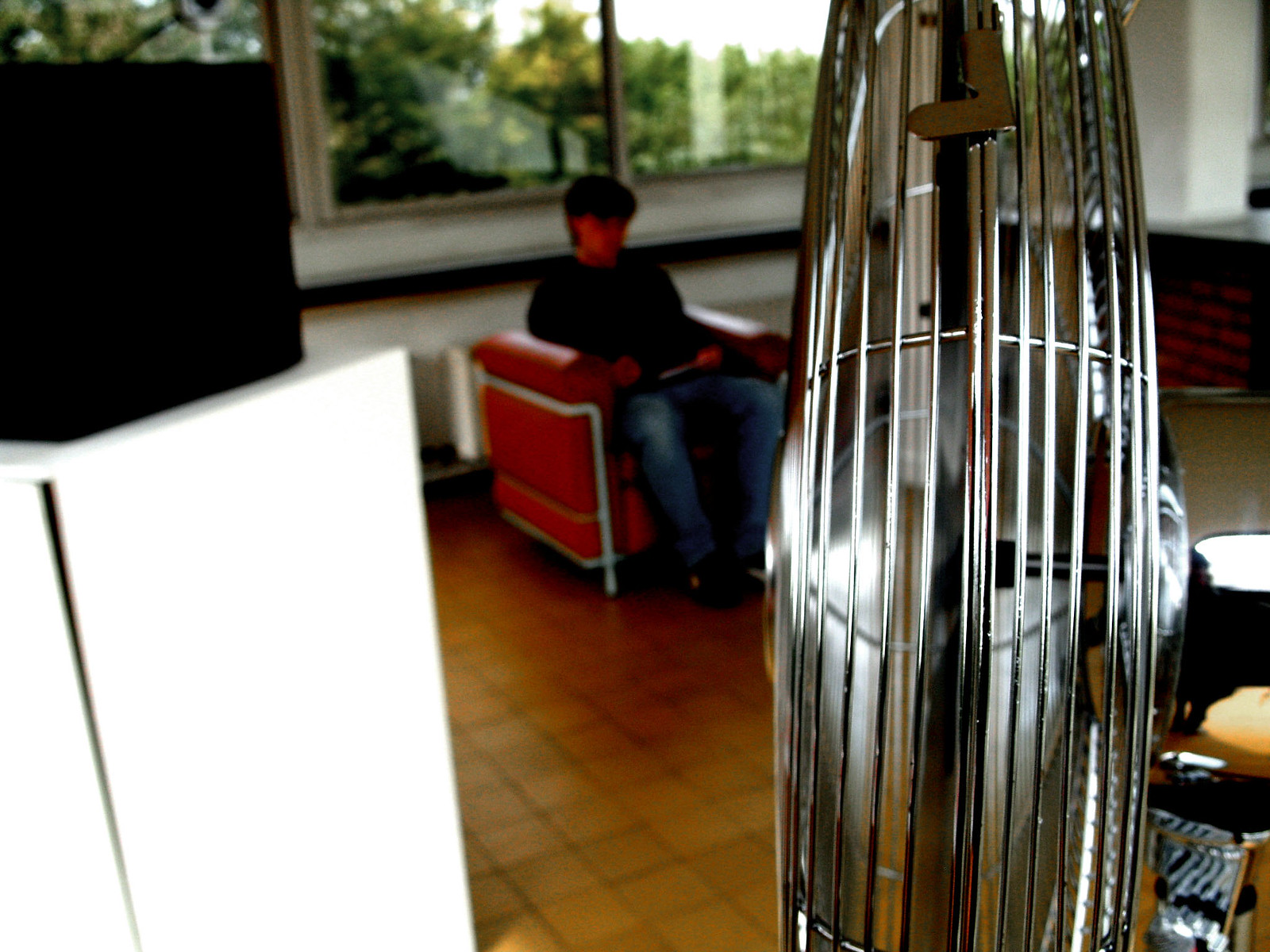This full-color photograph, taken indoors during the daytime, captures a well-lit scene that appears to take place inside a home or possibly a lobby waiting area. In the forefront, a metal electric fan is visible from the side, standing close to the camera lens. To the left of the fan is a white cabinet or table with a black appliance on top, potentially a microwave. The main focus of the photograph is a young man with brown hair, seated on a red chair that lacks any leg rest, suggesting it is not a recliner. He is wearing a darker long-sleeved shirt and blue jeans and seems to be engrossed in reading something held in his lap. The floor beneath him is covered in rather unattractive brown tiles, and the room's white walls provide a neutral backdrop. Behind him, large windows allow natural light to filter in, showcasing lush green trees outside, contributing to the room's bright and airy atmosphere. The setting might be a meeting room or a hallway, suggestive of a school or similar environment.